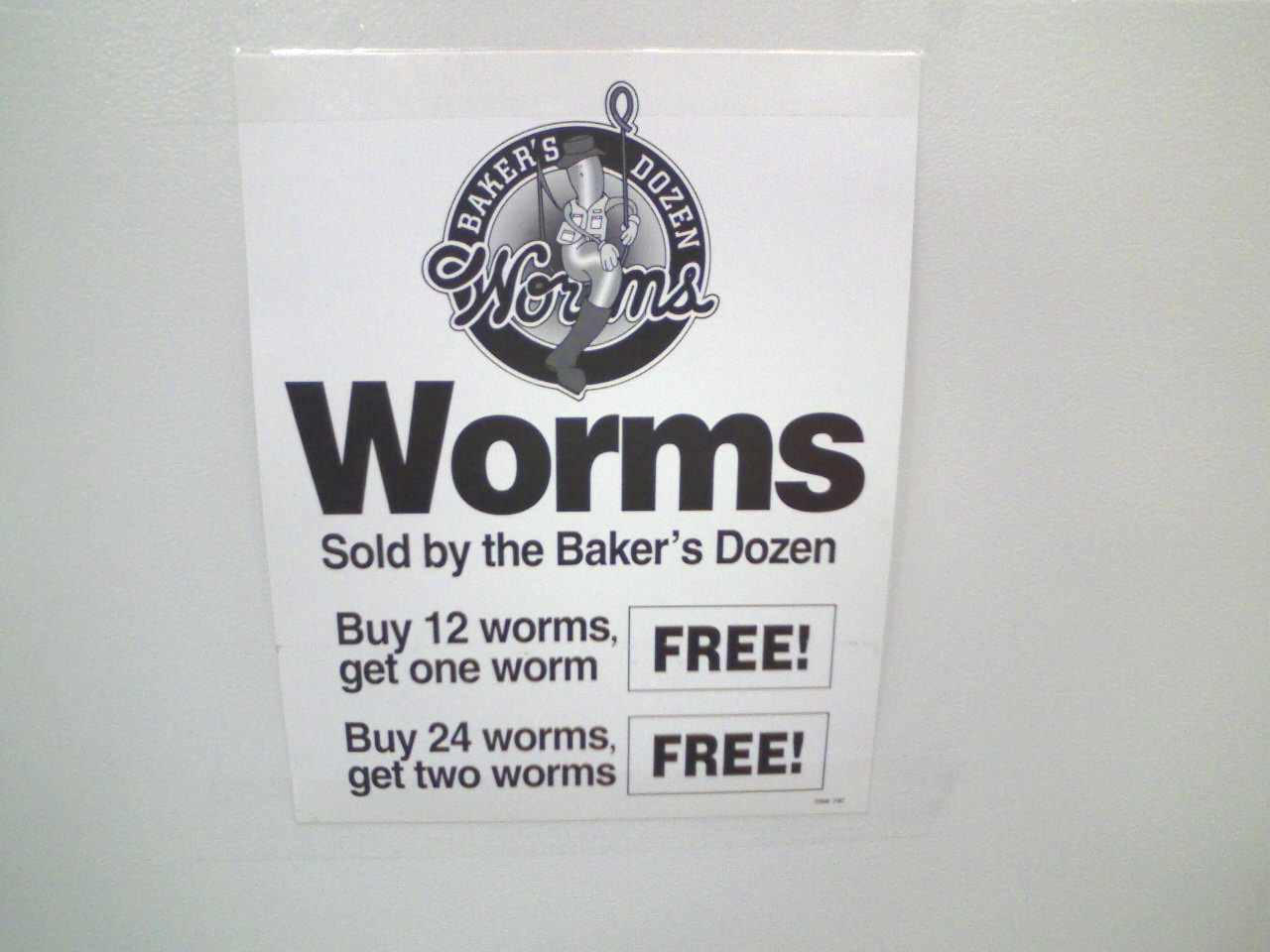The image, oriented horizontally, features a hand-crafted sign affixed to what seems to be the front of a refrigerator with clear vertical tape placed along its top edge. The sign is made of white cardboard and displays bold black lettering that reads "Baker's Dozen Worms." At the center, there is a whimsical illustration of a stylized worm dressed in a fisherman’s jacket and waders, perched on a hook with a circular bullseye backdrop. Beneath the illustration, the word "Worms" is prominently displayed in large, bold black letters. Following this, the text in a smaller, yet still bold, typeface states, "Sold by the Baker's Dozen." Additional promotional details are listed: "Buy 12 worms, get one worm free," and further below, "Buy 24 worms, get two worms free."